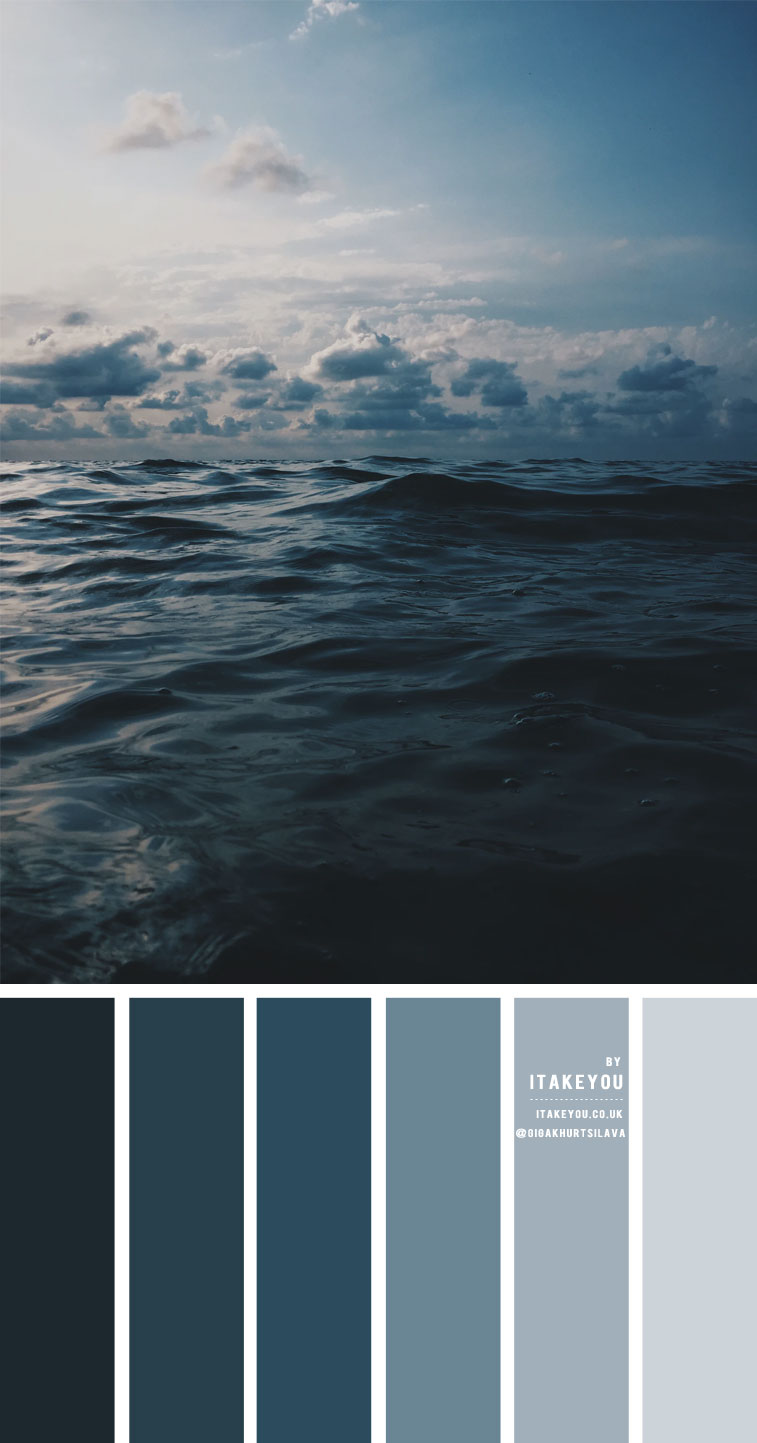The image is a vertically-oriented photograph of the ocean, almost like a portrait. At the top two-thirds of the image, dark, choppy waves of the sea dominate under a partly cloudy sky. The clouds are thicker and more concentrated towards the horizon, with the sun hidden behind them, casting a gloomy atmosphere over the scene. The sky's hues fade from a brighter light blue at the top to a darker shade towards the right corner. The bottom third of the image features a gradient palette of six distinct shades, transitioning from an extremely dark blue to a pale gray. These colors provide a stark contrast to the sea above, depicting a range of bluish-gray tones. Overall, the photograph captures the ocean's dynamic surface and the subdued, cloudy sky above, complete with various shades of blue that transition seamlessly from the natural scene to the color samples below.